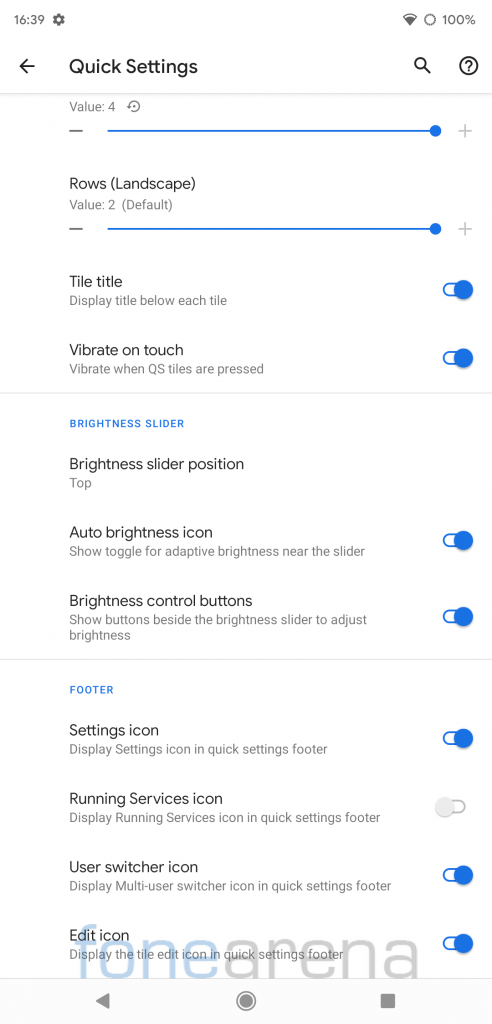The image appears to be a screenshot taken from a smartphone, showcasing the “Quick Settings” menu in detailed view. 

- The top of the screen displays the current time (16:38) and a gear icon in the upper left corner. To the right, there are icons for Wi-Fi signal and battery percentage (100%).
- Below the status bar, an arrow pointing left alongside the title "Quick Settings" is visible, with a search icon and a circular question mark icon to the right.
- The first section below this contains a slider labeled "Value," presented as a blue line with a dot at the end, illustrating its level. 
- The next line states "Rows (Landscaper)" followed by "Value 2", which also has a blue line with the dot positioned at the extreme right end.
- Further down, there is a setting titled "Tile Title" with the description "Display title below each tile," and next to it is a blue toggle-on button.
- The following option is "Vibrate on touch" accompanied by a description "Vibrate when OS tiles are pressed." This also has a blue toggle-on button.
- A blue brightness slider is marked, indicating its adjustability level. It is accompanied by the label "Brightness Slider Position Top," and offers options such as "Auto Brightness Icon," "Show," "Toggle," or "Adaptive Brightness." Alongside the slider, there is another blue toggle-on button.
- The "Brightness Control buttons" option is visible with an accompanying blue toggle-on button. 
- The section beneath this is headed "Footer" in blue text. 
  - "Settings Icon" is listed first with a toggle-on button.
  - "Running Services Icon" is listed next and is currently toggled off.
  - "User Switcher Icon" follows, toggled on in blue.
  - Lastly, the "Edit Icon" is also shown as toggled on in blue.

This meticulous layout clearly describes the different customizable settings within the Quick Settings menu.